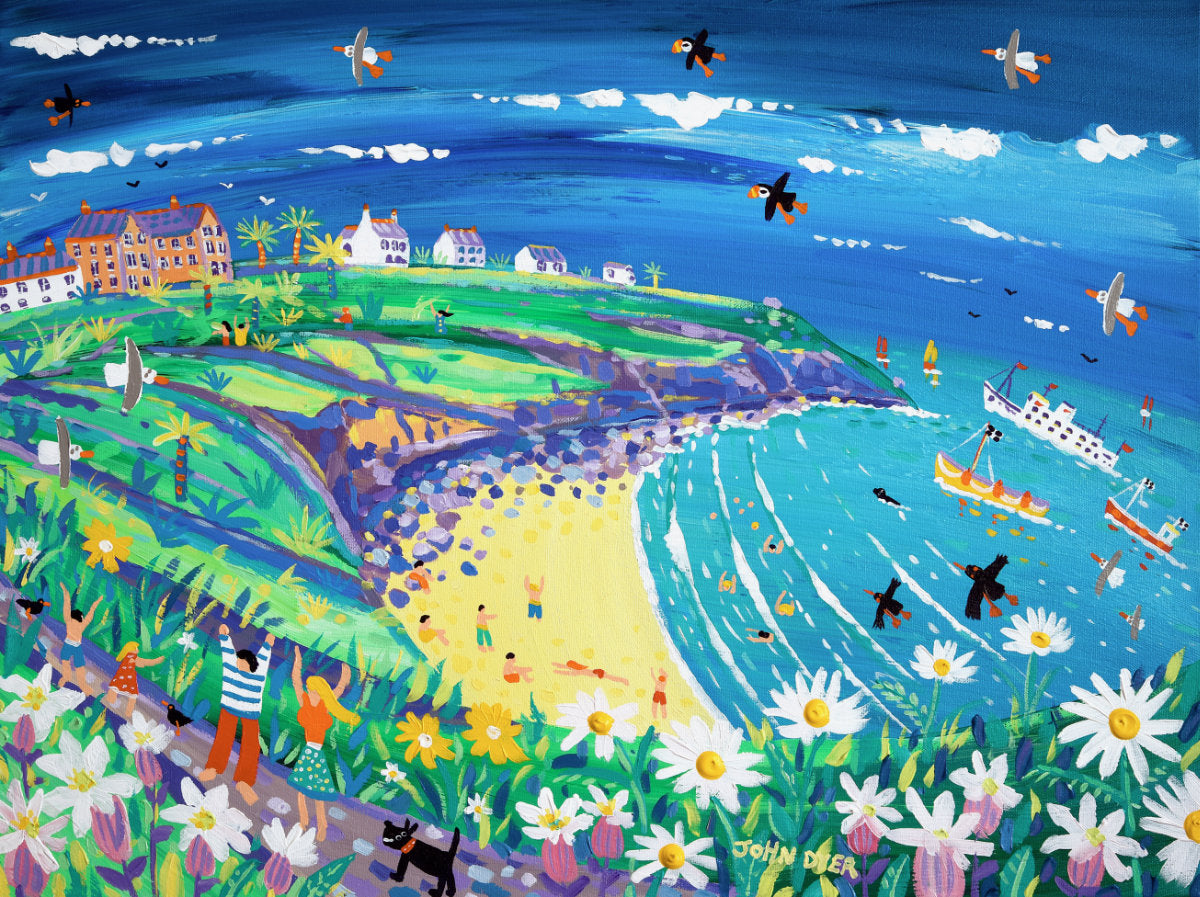The painting depicts a vibrant, aerial view of a diverse landscape. On the left side, lush green fields dotted with five white houses with purple roofs and two orange houses with purple roofs spread out across the countryside. At the bottom of the image, a road winds through, populated by various people and a black dog wearing a red collar. Alongside the road, colorful flowers with white petals and yellow centers burst into bloom. Black birds with white heads and orange beaks and feet, as well as white birds with grey wings and orange beaks and feet, fly gracefully in the sky and also dot the road. The central part of the image features a tranquil beach with people lounging and playing on the sand. The body of water, painted in beautiful ocean blue, hosts three ships and several swimmers. The sky above is a serene blue adorned with fluffy white clouds. The artwork also contains a faint text "John Deere," painted in yellow, positioned at the bottom middle, adding a final touch to this detailed and lively scene.